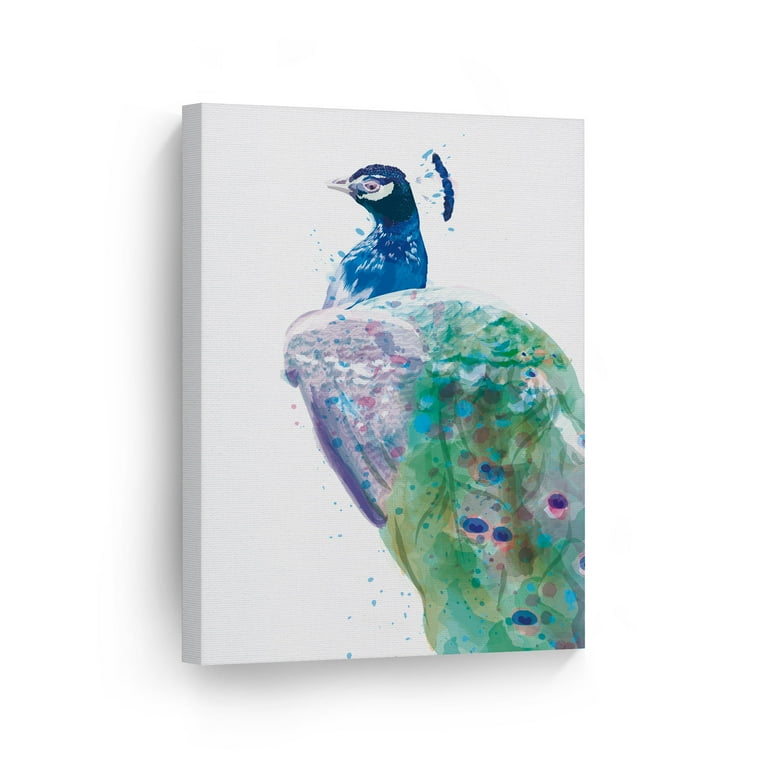This photograph captures a detailed painting of a peacock on a white three-dimensional canvas, which casts a shadow on the wall behind it. The peacock, a radiant composition of various colors, dominates the white, unpainted canvas. The head of the bird is primarily blue with a lavender eye highlighted by a white stripe underneath and a blue crest extending from the top. Its beak is a mix of white and gray. The peacock is oriented to the left, and its wings, which are tucked in and not fanned out, extend off the bottom right-hand corner of the canvas. The wings are adorned with shades of pink, green, and feature purple oval spots. Additionally, the back of the peacock showcases an emerald-green hue punctuated with dispersed dots of red and blue. The bird's upright posture and vibrant plumage create a striking centerpiece that vividly stands out against the minimalist, white backdrop.